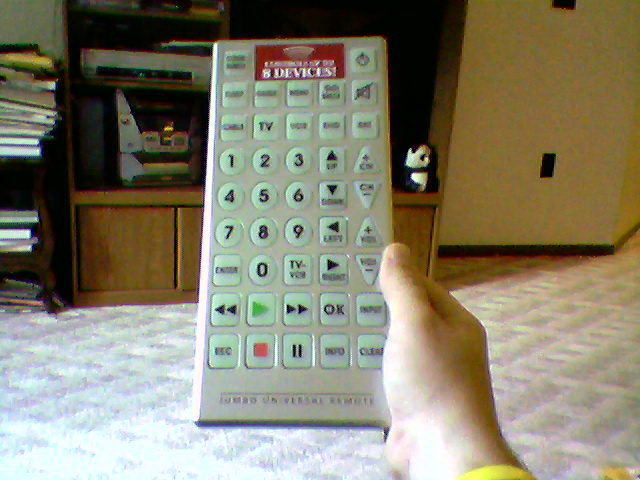The photograph depicts a low-resolution image centered around a large, rectangular, "Jumbo Universal Series" remote control held vertically by a right hand with a visible thumb emerging from a yellow shirt sleeve. The remote, which features numerous labeled buttons including numeric keys, channel and volume controls, and playback options, has a noticeable red badge at the top middle, partially readable as "B devices." In the backdrop, there is a beige carpet with a diamond pattern and an entertainment center draped in a brown TV console with possibly four drawers at the bottom. Atop the console lies a silver stereo system receiver underneath a DVD or VCR player. On the right side of the console, a small statue with black hair and a likely black cloak, reminiscent of Peter Lorre, is seen, although some suggest it resembles a panda statue. On the far left, a separate dark brown to black table, cluttered with books and papers on top, is partially visible, with more papers stored in the cupboard space below. The scene is bordered by white, slightly yellowish-ivory walls.